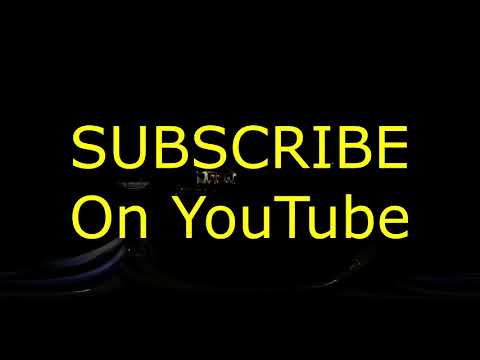The image is a color digital photograph with a predominantly solid black background, presenting a slightly rectangular shape. Despite the darkness, faint details are visible, including subtle gray curves on the left and faint, indiscernible shapes that might suggest people or objects. The primary feature is centered bright yellow text composed of two lines. The first line, in all capital letters, reads "SUBSCRIBE," while the second line says "ON YOUTUBE," with the words "YouTube" having a capital Y and T. These lines of text are neatly aligned on top of one another. Surrounding the text are speckles of white light, which further obscure the already shadowed and indistinct background, making specific details difficult to perceive.